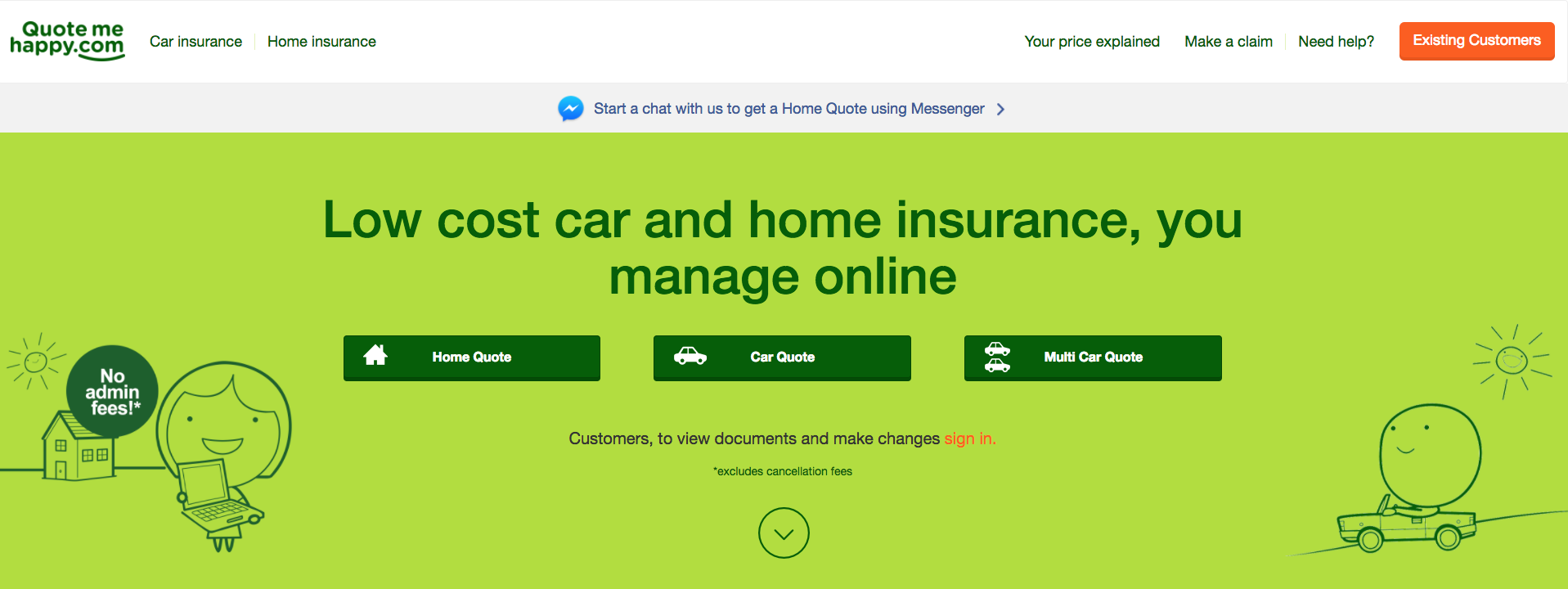The screenshot showcases the homepage of the mehappy.com website. In the upper left-hand corner, the website's name is prominently displayed. Adjacent to it, the top navigation bar features several options: "Car Insurance" in green font, "Home Insurance," "Your Price Explained," "Make a Claim," and "Need Help."

Located towards the right side of this navigation bar is an orange button labeled "Existing Customers" in white font. Below the navigation bar, a horizontal gray bar spans the width of the page, with centered text that prompts visitors to "Start a chat with us to get a home call using messenger."

Further down, a green banner stretches across the entire width of the page, displaying the message "Low-cost car and home insurance. You manage online." in green font. Below this banner, there are three buttons for obtaining quotes: "Home Quote" on the left, "Car Quote" in the center, and "Mail Multi-Car Quote" on the right.